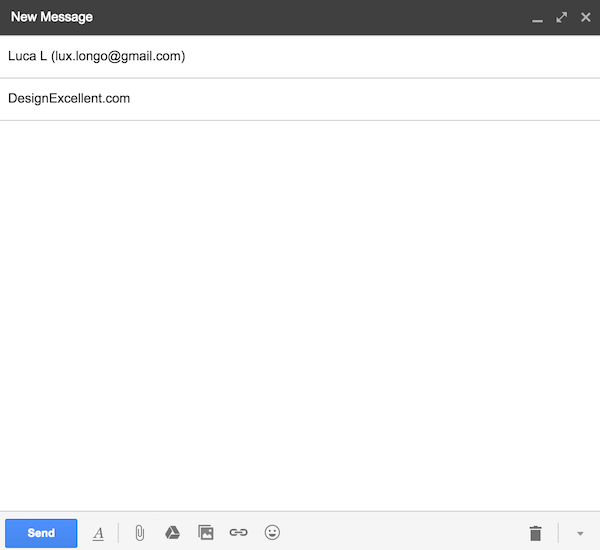An open email is displayed on a computer screen with a predominantly white interface. At the top, a black bar stretches across the screen, containing "New Message" in white, left-aligned. On the far right of the bar are three icons: a white "X" for closing the email, a double-headed arrow for expanding, and an underscore for minimizing the window.

Below this black bar is the address field, where the recipient’s information has been filled in: "Luca L." followed by the email address in brackets, "lux.longo@gmail.com." A thin gray line separates this section from the subject line, which reads "designexcellent.com."

Another gray line separates the subject line from the body of the email, which is currently blank. At the bottom of the screen, a pale gray bar contains several functional buttons. On the bottom left is a blue "Send" button. To its right, an italicized "A" over an underscore represents the formatting options. Next are icons for attaching files: a paperclip for attachments, followed by icons for Google Drive, photos, inserting links, and emojis. On the far right of this pale gray bar are the bin icon for deleting the draft and a drop-down menu for more options.